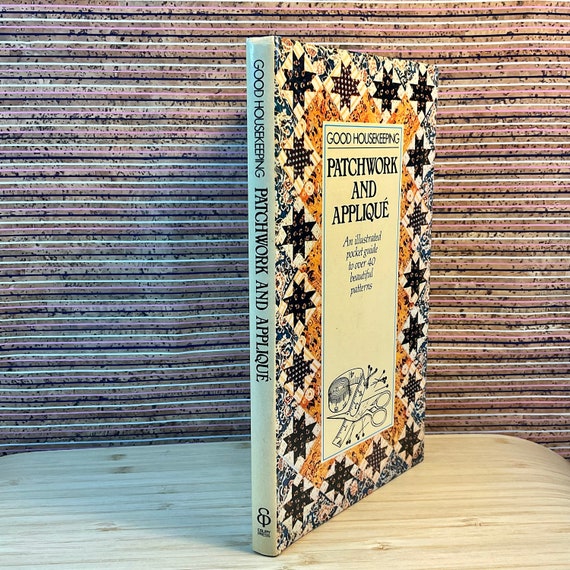The image presents a detailed view of a book standing upright on a light wooden table, positioned centered in the frame. The spine of the book runs vertically, while the cover is angled slightly to the right. The book is titled "Good Housekeeping: Patchwork and Appliqué". The cover features vibrant colors, including black, yellow, blue, and white, with various patterns indicative of patchwork. The book's cover text describes it as "an illustrated pocket guide to over 40 beautiful patterns," and includes illustrations of patchwork tools such as a ruler, scissors, and needles. In the background, the top three-fourths of the image showcase a back wall adorned with pink, brown, and white hues, while the bottom fourth consists of the wooden table. The photograph appears to be taken indoors, with a focus on highlighting the book's intricate design and craftsmanship.